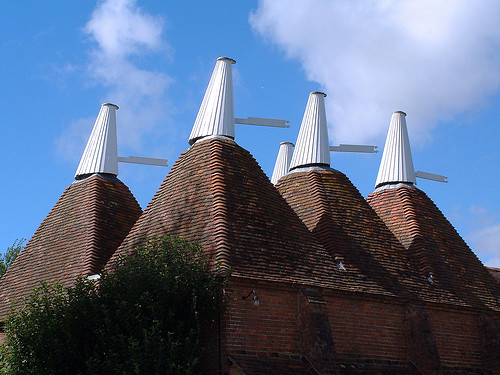The image depicts a distant view of a distinctive building under a vibrant blue sky with sparse, puffy white clouds—one resembling a dragon on the left and another cylindrical shape on the right, the latter being larger. Dominating the scene are five imposing, steeply-peaked roofs covered in brownish-red tiles, each pinnacle adorned with a white, corrugated, circular pyramid structure that appears to serve as a ventilation feature. These features, potentially chimneys, lend an industrial touch to the otherwise rustic structure. The building's façade is composed of brown to dark white bricks, adding to its robust appearance. At its base, green trees and shrubs embellish the left side of the frame, indicating a verdant spring or summer setting. The image is characterized by a serene and clear day, showcasing the interplay of natural and architectural elements harmoniously.